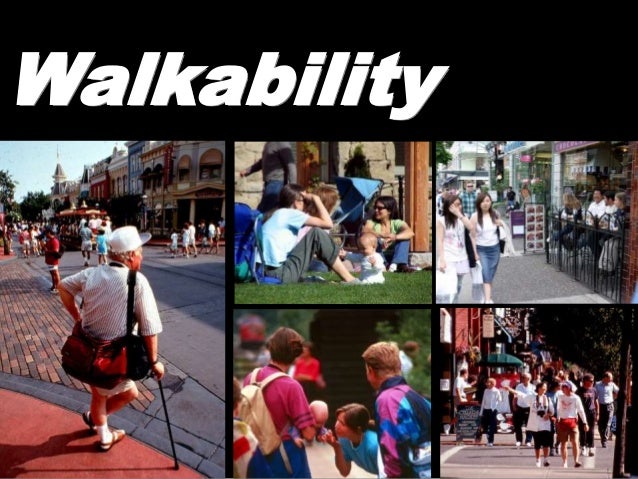The image features a vibrant, colorful photo collage framed by a black banner at the top with the word "Walkability" prominently displayed in white letters. The collage comprises five distinct photographs, each capturing various aspects of urban life. 

On the far left, there's a tall, narrow photo of a man standing with his legs crossed, leaning on a black cane. He is dressed in a white baseball cap and a matching shirt, with a red duffel bag slung over his shoulder. He appears to be gazing at a street filled with buildings and pedestrians in the background.

To the right, a grid of four smaller images is arranged in a 2x2 layout. In the upper-left of this grid, a family is seen sitting on green grass next to a stroller, enjoying a serene outdoor moment. Below this, another group is depicted where one individual bends down, engrossed with a baby held by another person. 

The upper-right image of the grid shows two women walking down a lively street, adjacent to an outdoor café, suggesting a bustling, vibrant neighborhood. The bottom-right photo mirrors this lively ambiance with another pair of women walking down the street, surrounded by a multitude of other pedestrians indicating a busy urban environment.

The entire collage is rich with a palette of colors—reds, whites, blacks, blues, purples, and greens—capturing various scenes drenched in natural light, which enhances the clarity and liveliness of the images. The overall impression is one of an inviting, walkable city where people enjoy both community interactions and their daily strolls.